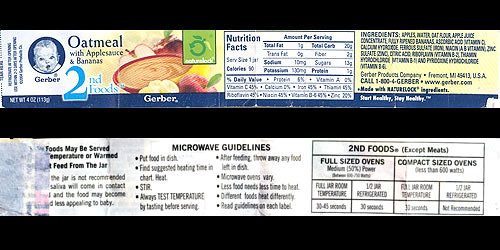This image features two distinct labels from a Gerber oatmeal with applesauce and bananas, second foods jar, set against a black background. The overall image is approximately two and a half times wider than it is tall. On the upper left of the image, there is a prominent Gerber label showcasing the Gerber baby logo, with text reading "Oatmeal with Applesauce and Bananas" and "Second Foods" written in blue. Adjacent to this, moving to the right, is a white nutrition facts section with dark lettering. Further right is a list of the ingredients. 

In the lower portion of the image, there is a second label that appears worn and partially obscured on the left side. This label suggests that the food can be served at different temperatures and includes more details on feeding instructions. To the right of this, it provides microwave guidelines, specifying cooking times for both full-sized and compact ovens. The term "Second Foods" is also mentioned again on this label, reinforcing the product's identity. Overall, the two labels together comprehensively display crucial product information, nutritional data, and preparation guidelines.